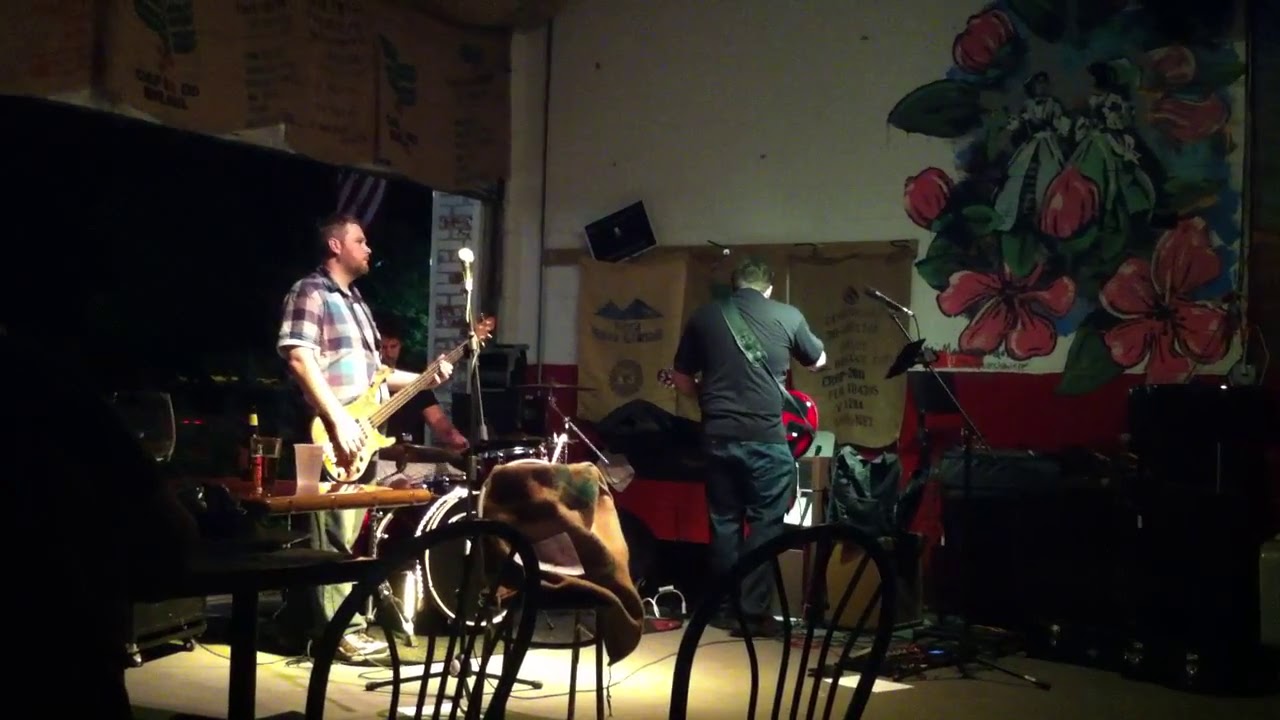The image is an indoor photograph of a band mid-set. Central to the picture is a man with dark hair wearing a plaid shirt, holding a yellow guitar. To his left, partially shown, is another man with a red guitar strapped to his front, dressed in dark colors. Chairs and tables are scattered in the foreground, likely places where an audience could sit to watch the performance. Behind the men is a long black screen and large brown boxes. The walls are adorned with paintings and graffiti, including a prominent piece with red and green flowers. Burlap sacks with unreadable text are also hanging on the beige wall to the right and at the top of the other wall.